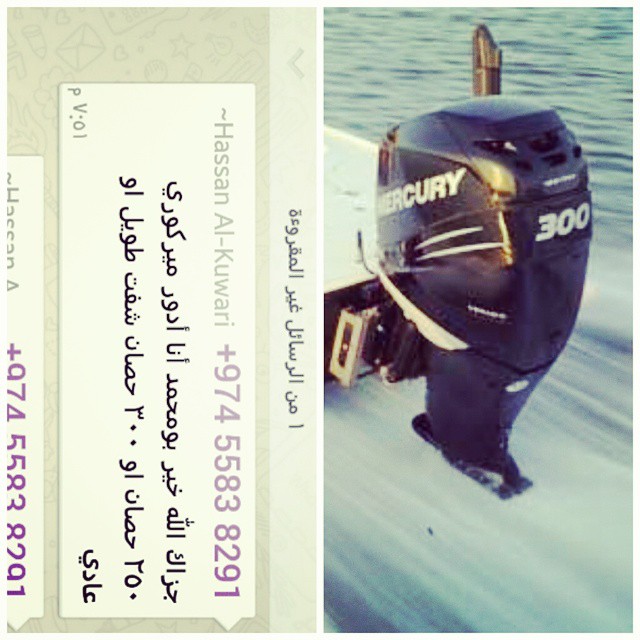The large square image is divided into two distinct halves. The right half features a detailed image of a black boat engine with the brand name "MERCURY" in bold white letters and the number "300" prominently displayed. The engine is mounted on a white surface, likely a boat, and in the upper-right corner, gentle ripples on the water suggest the boat is in motion. On the left half of the image, a vertically oriented white rectangle contains a message with a gray, subtly decorated background featuring stars, hearts, and envelopes. The text within this rectangle includes the name "Hassan Al Khawari" printed in gray, followed by the phone number "+974-5583-8291" in purple. Below, there are two lines of text in a non-English language, possibly accompanied by a signature, and the code "PV: O1" appears in the lower right corner of the rectangle.